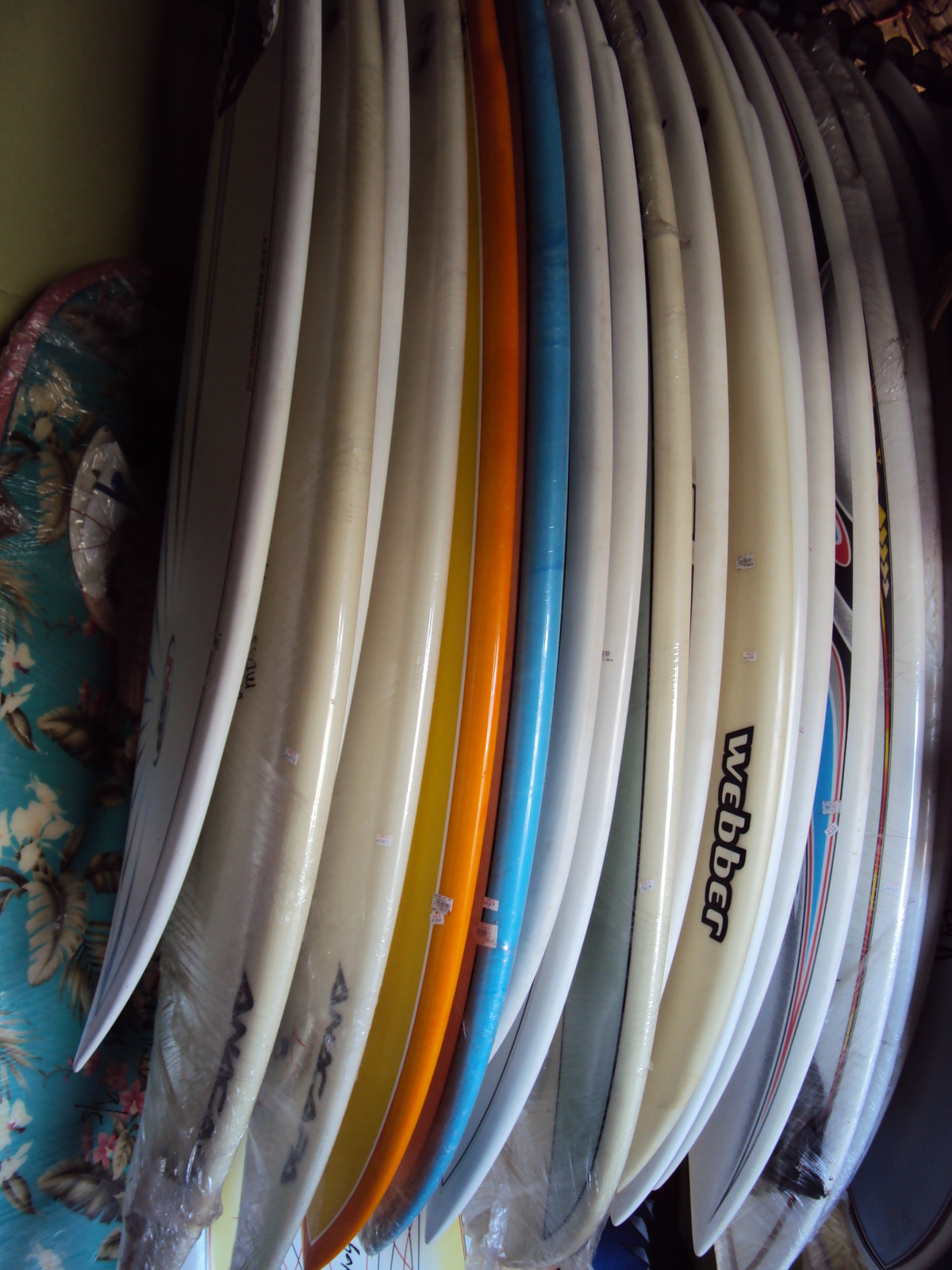This photograph features an array of surfboards and body boards viewed from the top down, closely grouped together, some wrapped in cellophane. The boards vary in size, length, and branding, with some notable brands including Weber on a white board and Anara. The surfboards exhibit a range of colors such as orange, blue, light yellow, and some with stripe patterns. One particular board on the outside showcases an orange edge with a thin white line, merging into a yellow center. In the background, a boogie board decorated with Hawaiian floral patterns leans against a dark wall, which adds to the shadowy ambience of the photograph. The image is colorful but shaded, with light reflecting off the bottom parts of the boards, creating a striking contrast against the darker upper section.